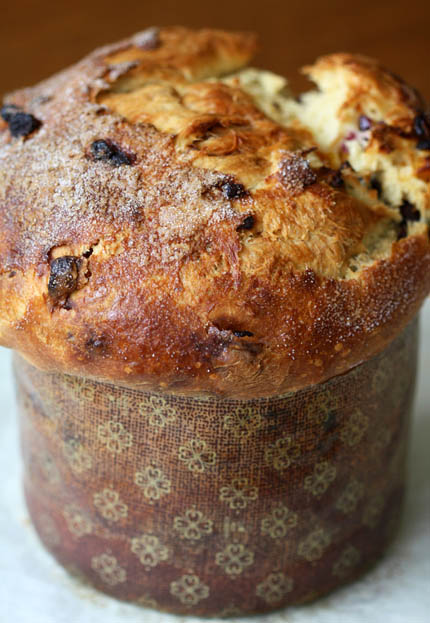This close-up photo captures a golden brown muffin, potentially flavored with blueberries, cranberries, or chocolate chips, showcased atop a white table or plate. The muffin, which could also be mistaken for bread due to its risen top and circular shape, is wrapped in a unique, fibrous holder resembling woven cloth rather than traditional paper. The holder is a natural brown color adorned with a pattern of tan flowers, each resembling a four-leaf clover. Speckled throughout the top of the muffin are small, dark bits of fruit or chocolate, suggesting a freshly baked texture with a soft, inviting interior. The background of the image is a contrasting, earthy brown, further highlighting the ornate details and appetizing appearance of the muffin.